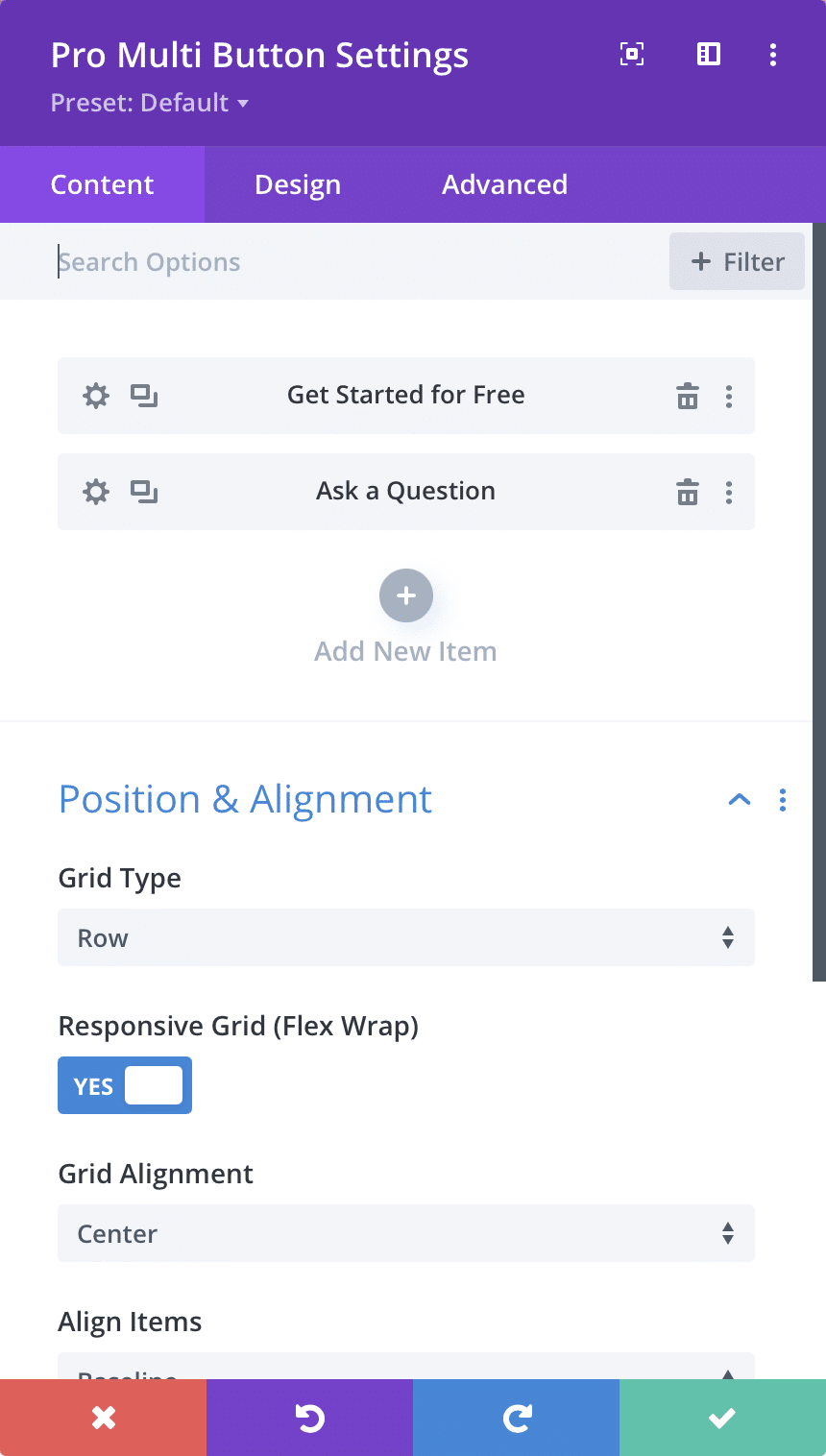The image in question is in portrait format, boasting vivid colors. It appears to be a screenshot captured from a mobile phone, depicting a settings interface rather than an application. The upper section of the screenshot features a dark purplish banner that provides a sophisticated backdrop. At the lower segment, a palette of colorful buttons in red, purple, blue, and green displays various commands, adding a friendly and engaging touch to the interface.

The screen is labeled as "Pro Multi-Button Settings," with the current preset set to default, though customizable options are available. There are three primary tabs at the top of the screen: Content, Designer, and Advanced. The user is currently on the Content tab.

Beneath these tabs lies a search bar labeled "Search Options," facilitating a quicker search for specific settings. Further options include buttons for "Get Started for Free," "Ask a Question," or adding a new item.

Underneath these initial options is a section dedicated to "Position and Alignment." This section provides various customization choices like grid type, which is currently set to "Row," with the implication that other configurations such as columns might be selectable. Other options in this section include "Responsive Grid Flex Wrap," which can be toggled to 'yes,' and settings for "Grid Alignment," which are defaulted to 'centered' and 'align items.'